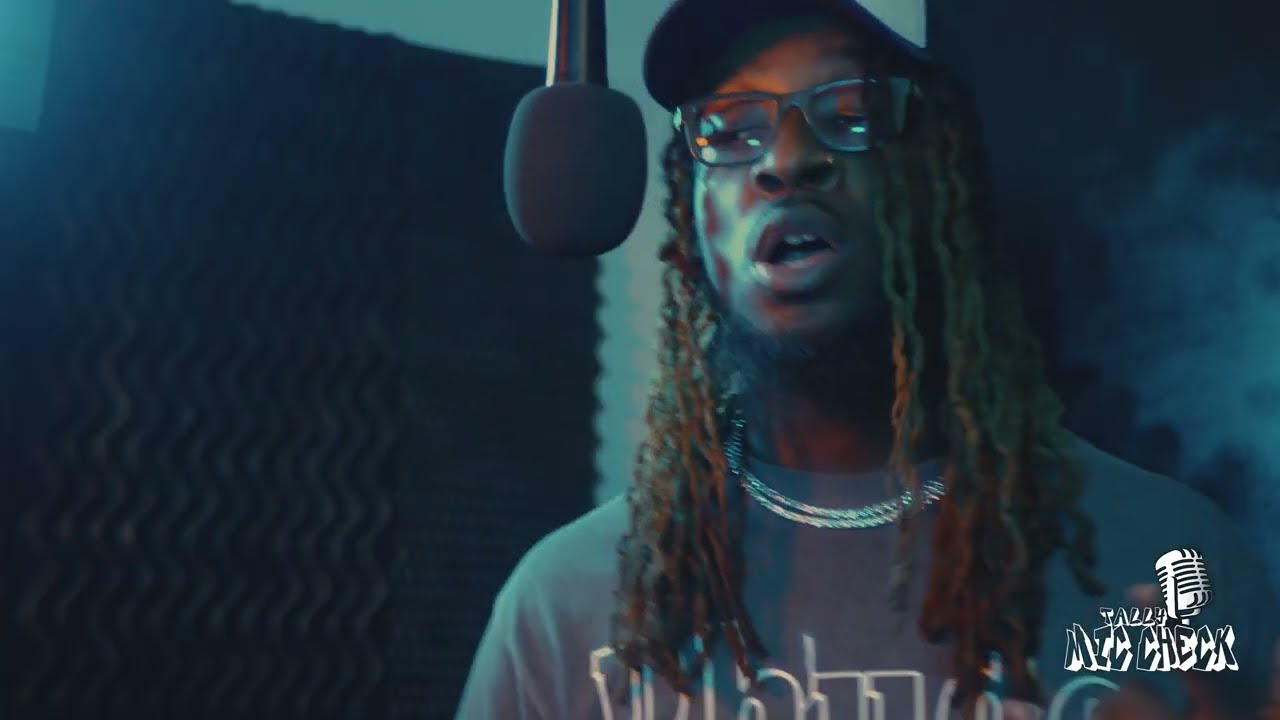The image captures a detailed scene inside a recording studio. At its core is a black man with long dreadlocks, their tips colored blonde or light brown, which fall to about chest height. He wears dark-rimmed prescription glasses with a visible reflection, a grey t-shirt, and a hat. Around his neck, he sports multiple chains, described variably as silver or gold. The man is positioned almost centrally in the image, singing into a microphone that is suspended from above, directly in front of his face.

The backdrop features a blurred wall, likely outfitted with black soundproofing panels. This setting affirms the studio's purpose as a controlled acoustic environment. Colors in the image include shades of white, grey, black, and off-blue. In the bottom right corner, a logo appears, depicting a microphone alongside graffiti-style text that reads "Tally Mic Check." The overall style suggests that the picture was taken from the vantage point of someone observing a recording session.